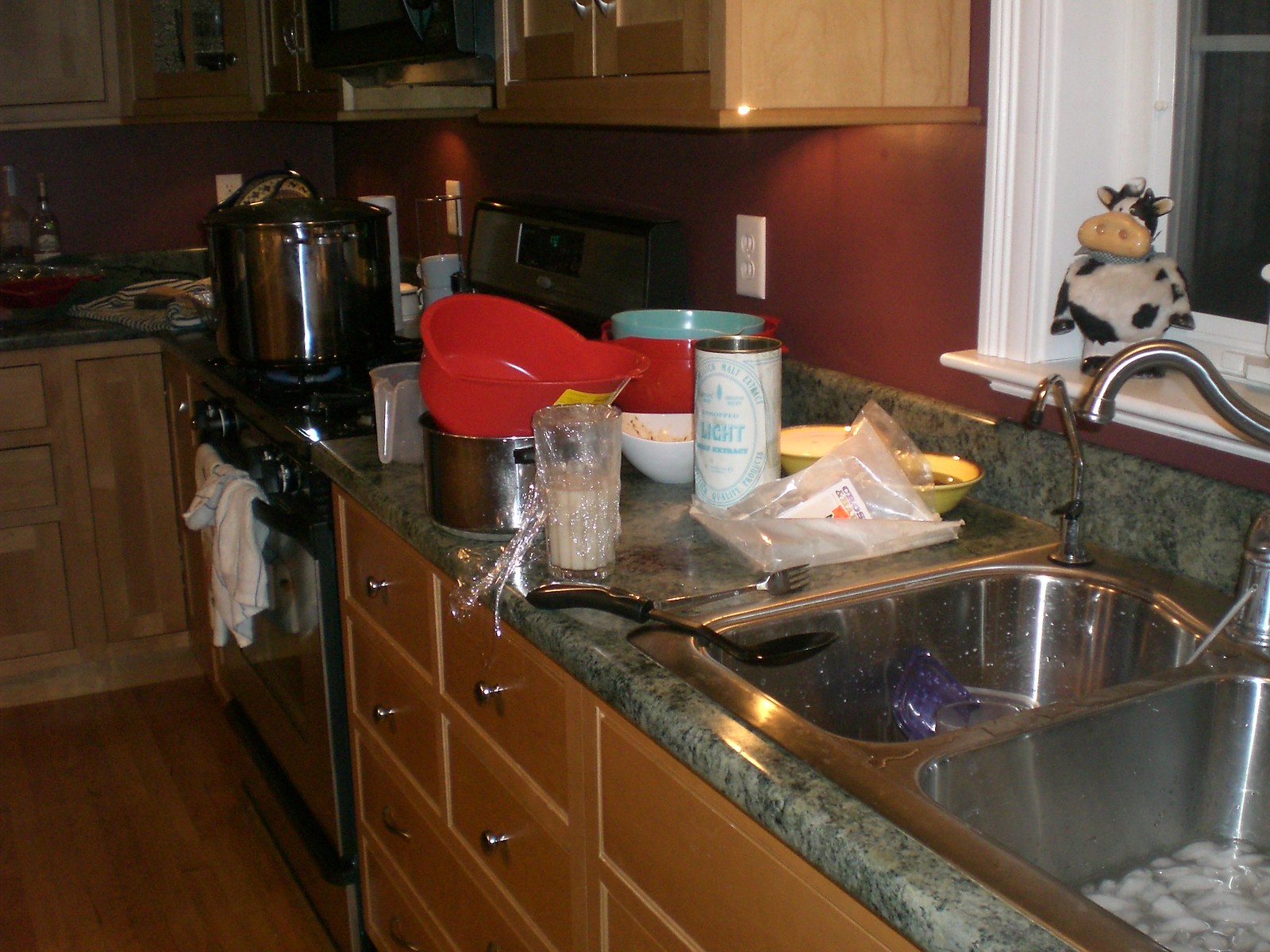A detailed caption of this color photograph captures a partial view of a kitchen interior centered around the countertop area. The photograph features the upper right corner of a window with white framing, revealing a small segment of glass adorned with a miniature cow figurine. The stainless steel sink is prominently visible, occupying about two-thirds of the image. The countertop showcases a greenish, marble-like pattern. Moving left from the sink, the surface is cluttered with various kitchen items, including silver and red bowls, containers, and a glass filled with a white liquid, covered with clear wrap. The lighting dims towards the upper left, casting shadows. The far end of the countertop reveals more clutter and slightly exposes the oven, identifiable by a rag hanging over its handle. Light wooden cabinets, partially visible at the top, complete the scene, offering a glimpse of the kitchen’s storage.